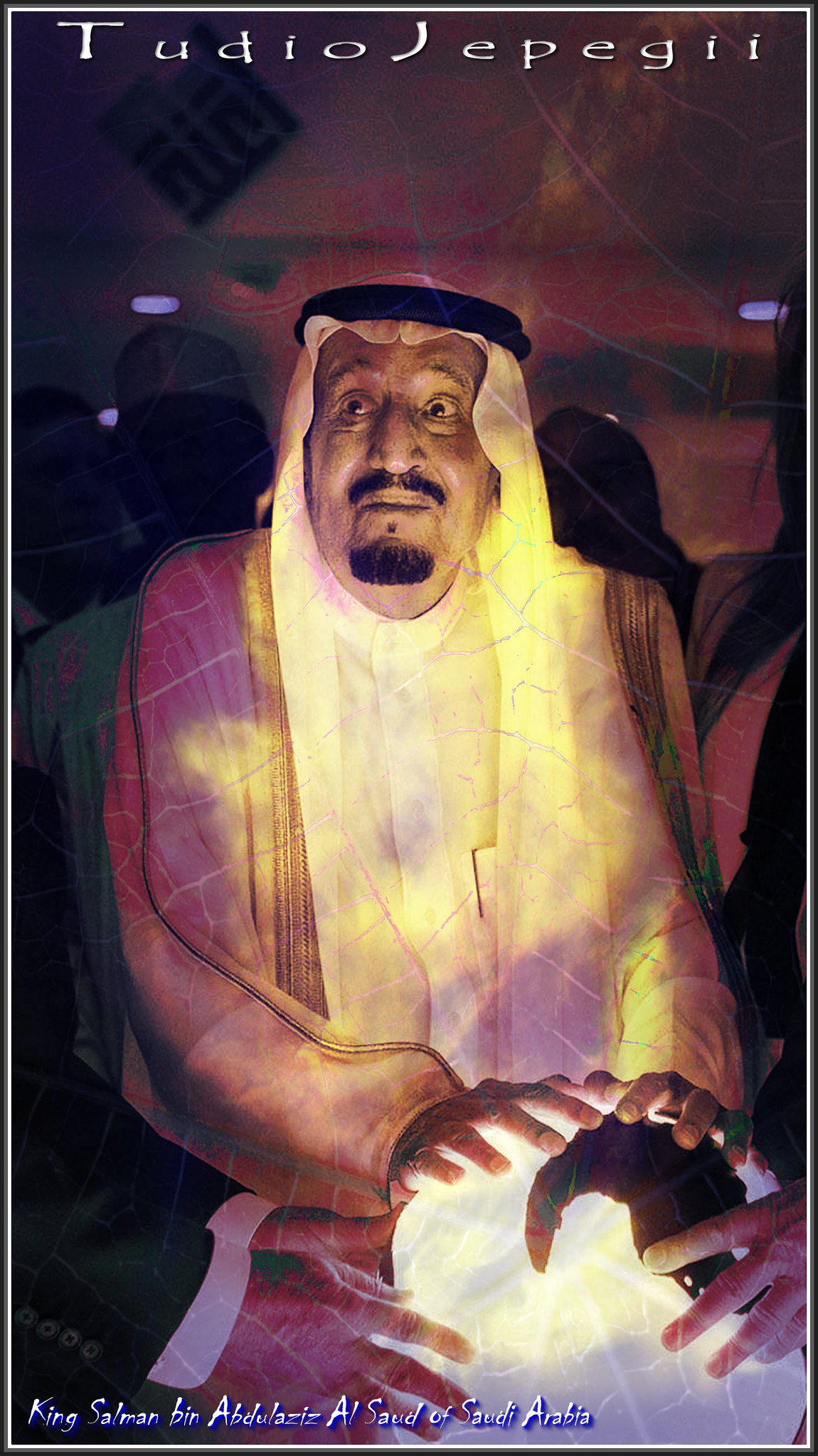This color photograph features King Salman bin Abdulaziz Al Saud of Saudi Arabia in traditional Saudi Arabian dress. He is wearing a white head covering secured with a black band and a light-colored robe. King Salman, who sports a goatee and mustache, is looking to his right while resting both hands on a glowing white orb. Visible to his left are the hands of another individual wearing a dark jacket with a white shirt, also touching the orb. To the right, another set of hands is barely visible, suggesting the presence of an additional person engaged in the scene. The background reveals a large room illuminated with ceiling lights. Text at the top of the image reads "Tudio Jepegi," and additional text at the bottom left, in white with a blue outline shadow, names him as King Salman bin Abdulaziz Al Saud of Saudi Arabia.